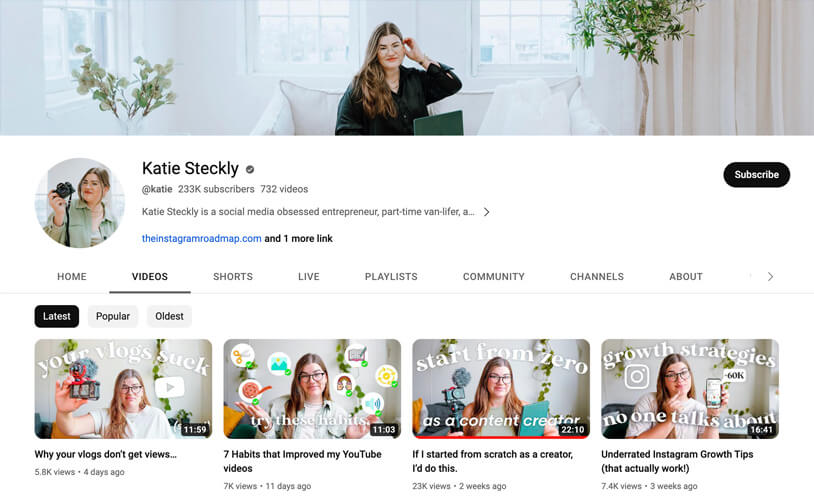The YouTube profile page of social media-obsessed entrepreneur and part-time van-lifer Katie Steckley is showcased. At the top of her channel, you see her name along with a large banner image featuring Katie comfortably seated on a sofa within a beautifully decorated house. Her profile picture, displayed as well, shows her confidently holding a digital camera, hinting at her passion for content creation. 

Navigating to the "Videos" section, options for various categories like Home, Shorts, Live, Playlists, Community, Channels, and About are available. The current focus is on her "Latest" videos, which are neatly sorted for easy exploration. The thumbnails for her recent uploads reveal a consistent theme: Katie appears in a neutral setting, dispensing valuable advice aimed at fellow content creators. 

Her latest video titles include "Why Your Vlogs Don't Get Views," "Seven Habits That Improve My YouTube Videos," and "If I Started from Scratch as a Creator, I'd Do This," which offer a blend of self-help and productivity tips tailored for aspiring YouTubers.